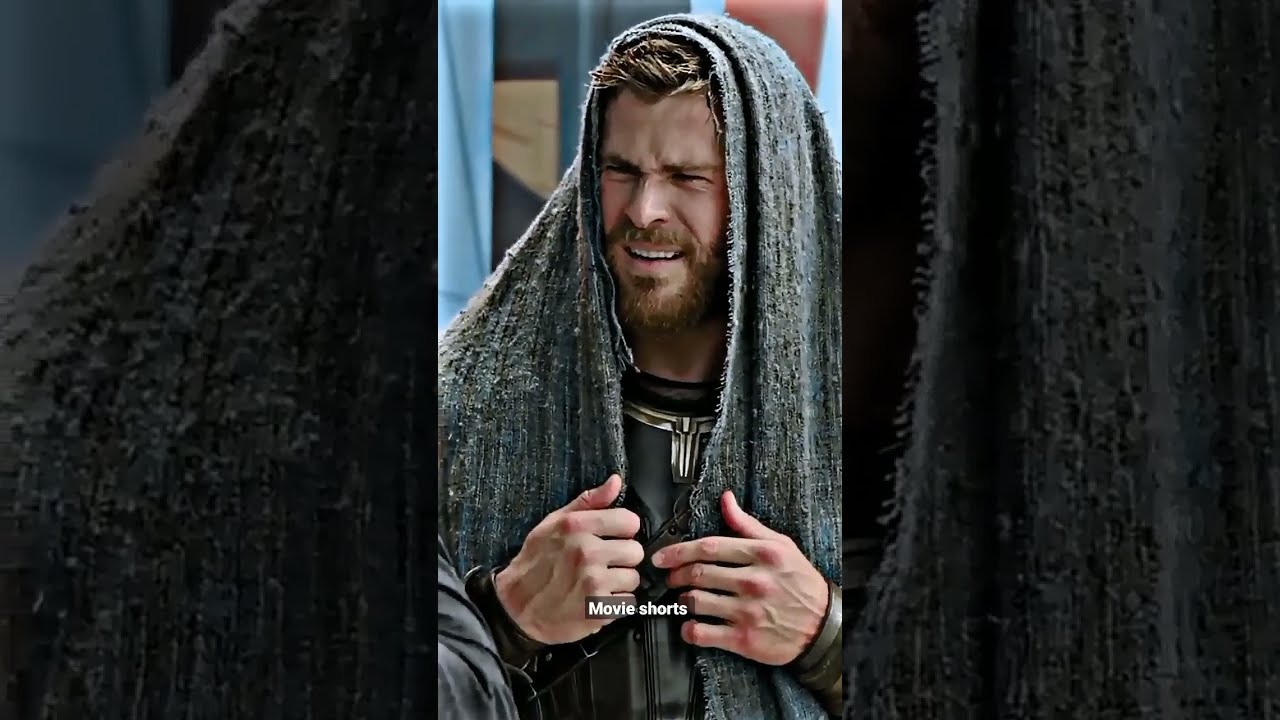The image is a horizontally rectangular snapshot, likely from a mobile device. It features a central, vertically rectangular portrait of a man who bears a striking resemblance to actor Chris Hemsworth. He is wearing an old-looking, dark gray hood that resembles a towel or head covering, giving him an appearance reminiscent of ancient times. His eyes, which are squinted, gaze to the left, and he has a brown beard and mustache with a bit of brown hair peeking out from under the hood. The man's hands are positioned near his chest, and between them is the text "movie shorts" in small white letters. He appears to be wearing some sort of dark armor or a gray and black top with decorative elements and a black collar. 

The background behind the man is indistinct, featuring shades of light blue, dark blue, and reddish hues, possibly resembling curtains. Flanking the central image, there are two wider, vertical rectangles that show close-up, faded-out sections of the left and right sides of the man's hood, creating a background effect. The lighting in the central image is better, while the sides exhibit a darker lighting.